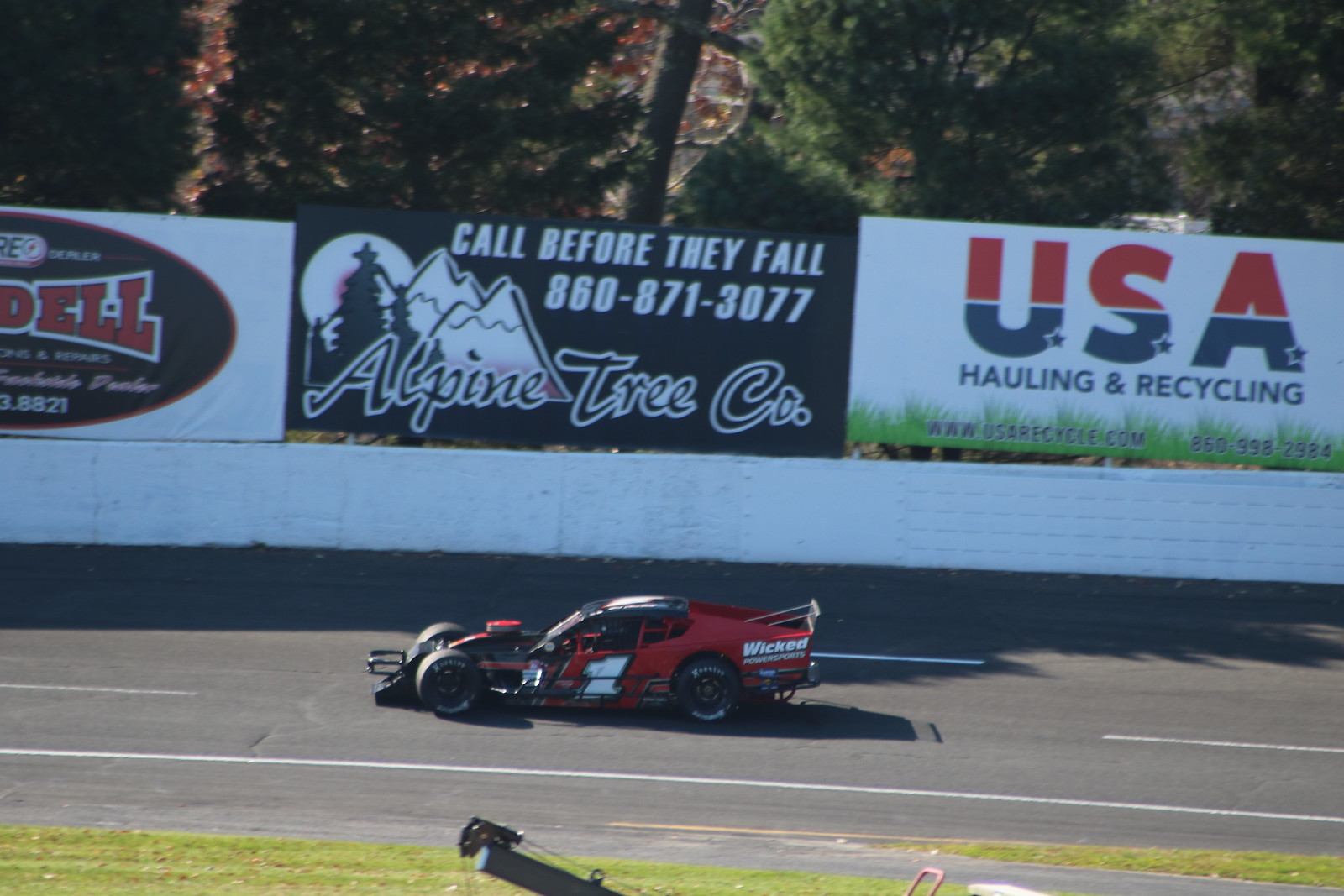This photograph captures a vibrant scene from a sunny day at a racetrack. Dominating the center of the image is a red NASCAR-style race car, adorned with a white number one on its side and the words "Wicked Power Sports" on its back. The car is moving to the left along a straight road flanked by a white stone wall that bears several advertising billboards.

The most prominent ads include one for the Alpine Tree Company, with the slogan "Call before they fall" and the contact number 860-871-3077. Adjacent to this is another advertisement for USA Hauling and Recycling, featuring red and blue lettering, a URL, and a phone number, with green grass depicted at the bottom. The wall and billboards create a distinct boundary around the track.

In the background, several tall trees and indistinct buildings peek above the wall, adding depth to the image. Shadows from the trees and the racing car provide a clear indication of the sunny weather. In the foreground, a piece of machinery is slightly visible, hinting at the infrastructural elements that support the racetrack environment.